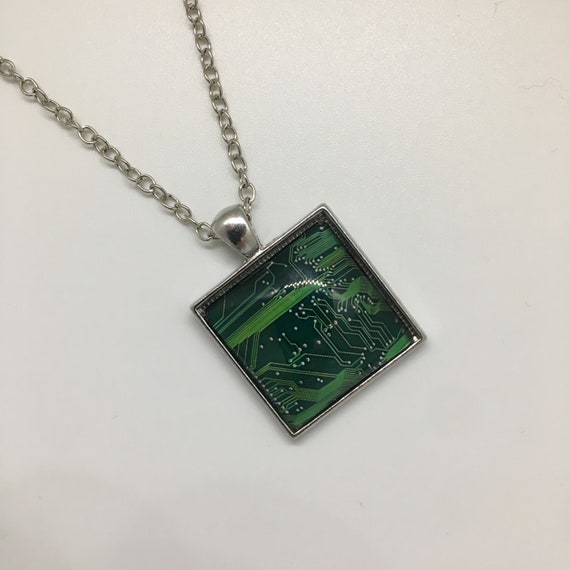This photograph captures a silver necklace laid on a white or light gray background. The necklace features a thin, circular link chain clasped to a unique pendant designed to mimic a piece of a circuit board. The pendant, which measures approximately an inch square, is encased in a thin, silver metallic frame. At its top, a wide, tapered silver loop secures the pendant to the chain, reflecting light subtly. The central focus of the pendant is a dark green microchip adorned with intricate circuitry patterns in lighter green and metallic white. The design includes silver-like dots resembling solder points and fine lines, reminiscent of a computer motherboard. This delicate and modern piece of jewelry fuses technological aesthetics with elegance, creating a striking visual effect.